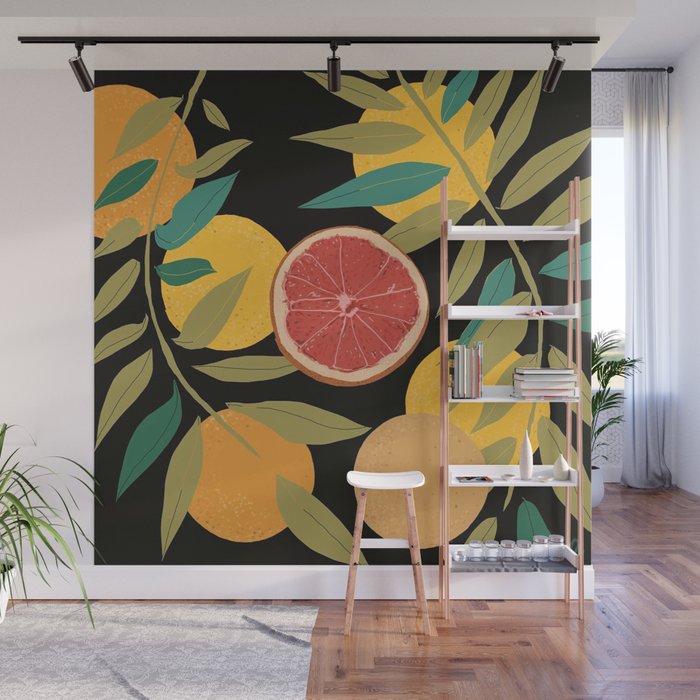The image showcases a meticulously designed indoor room featuring a captivating wall mural as the focal point. The mural, which almost occupies the entire wall, displays a sliced pink grapefruit at the center, surrounded by whole grapefruits and vivid leaves in a palette of green, yellow, and blue, set against a striking black background. The mural extends from the ceiling down to the baseboard and is illuminated by track lighting hanging from the ceiling— a horizontal black bar fitted with three directed fixtures.

To the right of the mural, there is a sleek, white bookshelf adorned with an assortment of books, vases, and candles. Adjacent to the bookshelf is a modern, four-legged stool with a white curved top. A beautiful gray rug with white patterns covers the left side of the wooden herringbone floor, which is a rich brown color.

The right side of the room features a window with floor-to-ceiling sheer white curtains, allowing light to filter softly into the space. In front of the window stands a potted green palm, contributing to the room's natural elements. A secondary planter with grass-like leaves is partially visible in the left corner of the image. The overall aesthetic of the room blends organic and contemporary elements, creating a balanced and harmonious interior.